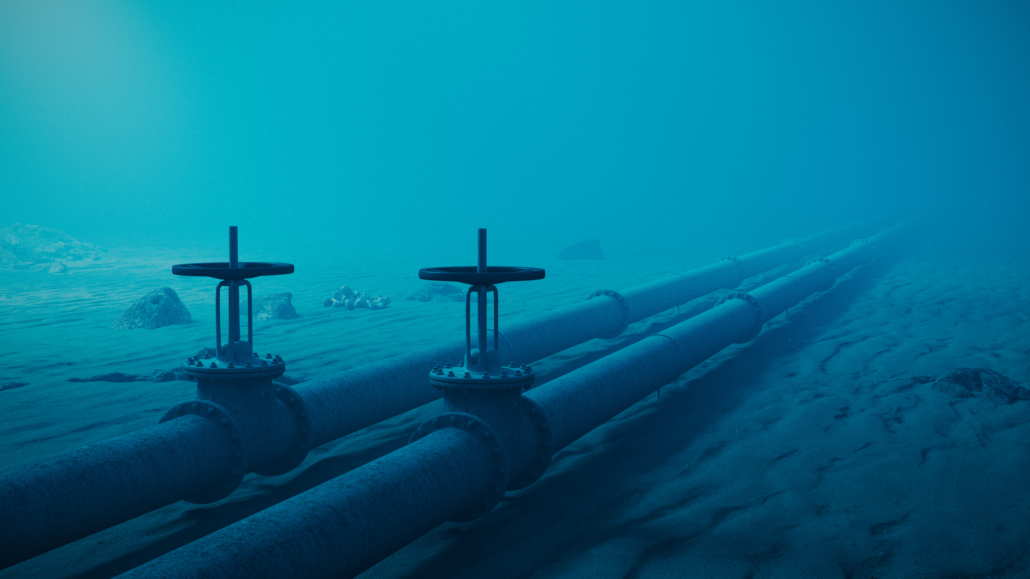The underwater photograph captures two large pipelines resting on a sandy and rocky ocean bed. The pipelines span from the lower left corner of the image, where they appear largest, stretching diagonally across to the upper right corner, diminishing in size with the perspective of distance as they fade into the clear blue water. Each pipeline is equipped with distinct valves characterized by riveted segments and wheel-like handles used for control, secured with visible nuts and bolts. The seabed around the pipelines features scattered rocks, further adding to the serene underwater landscape. The entire picture is enveloped in a cool blue tone, accentuating the clarity and depth of the underwater scene.